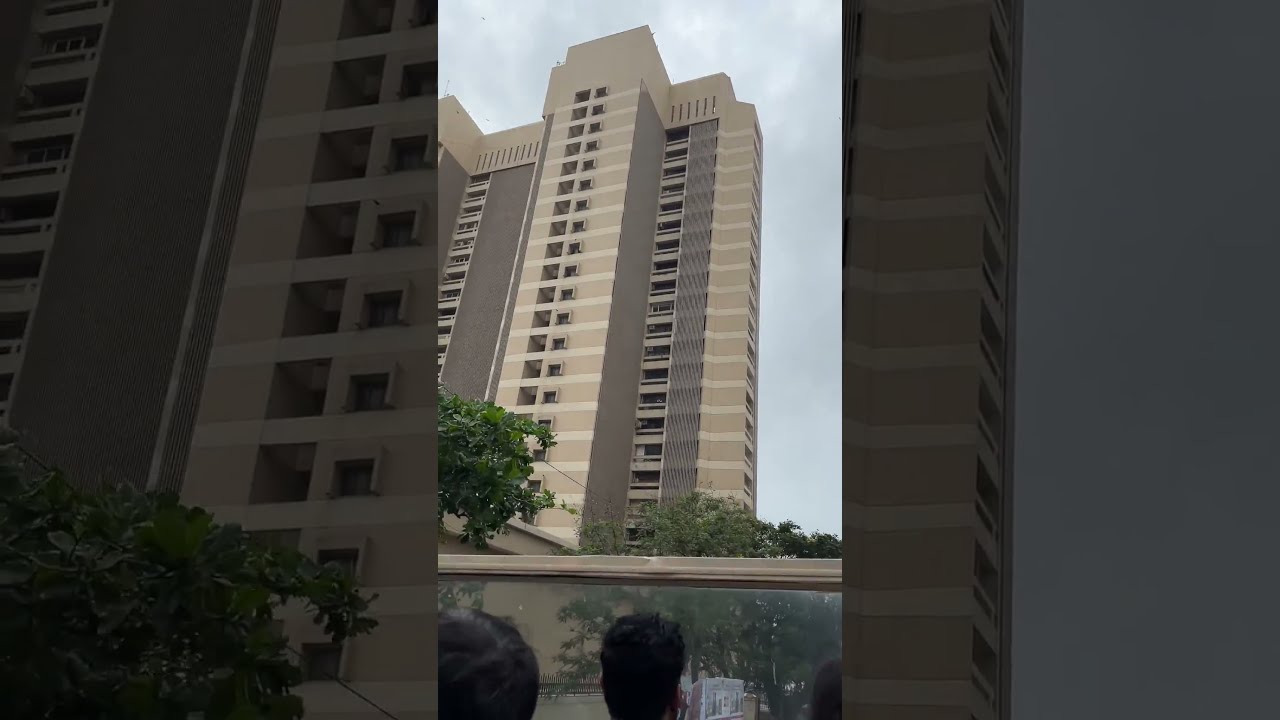This photograph captured from the upper deck of a double-decker bus features a bustling city scene dominated by a prominent traffic light showing green with a straight-ahead arrow. On the right side, a series of apartment buildings, each approximately four to six stories high, stretch diagonally across the image. These concrete edifices are interspersed with numerous windows and vary in color from beige to gray. Pedestrians walk along the sidewalk beside green leaf trees, while the asphalt road accommodates light poles and crosswalks. A man in a white shirt and khakis stands poised to cross the street. Above, the sky is shrouded in clouds, creating a gray overcast that hints at imminent rain. The bus's railing is visible in the frame, reinforcing the aerial perspective. Additionally, the aspect ratio suggests it might be a screen capture from a social media reel, bordered by grayed-out, enlarged segments of the main image.